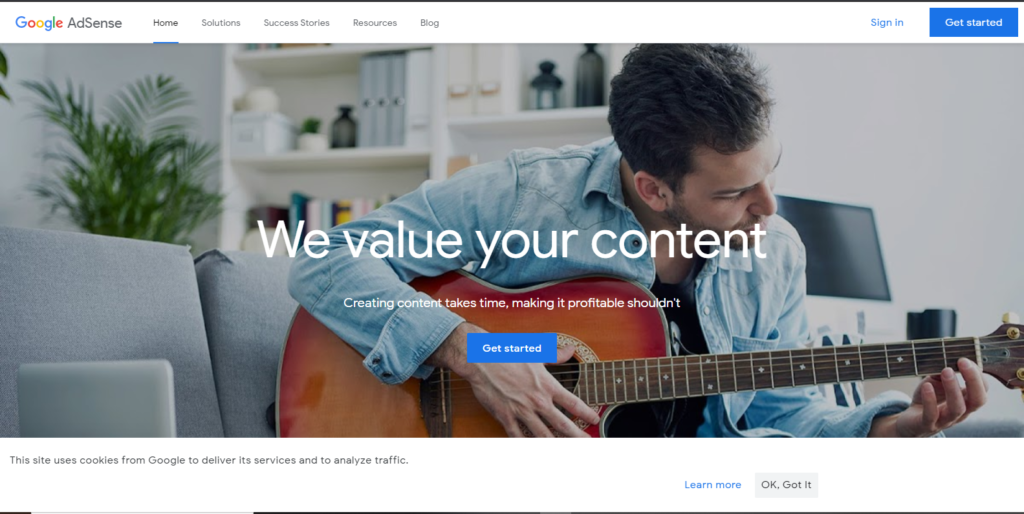This is a screenshot from the Google AdSense homepage. In the upper left corner, the navigation bar displays the text "Google AdSense," with "Google" in its traditional blue, red, yellow, and green colors, and "AdSense" in black. The navigation menu items include "Home," "Solutions," "Success Stories," "Resources," and "Blog." A blue line under "Home" indicates that the user is currently on the homepage. To the right, there are options to "Sign In" via a hyperlink and a blue button labeled "Get Started" in white text.

Below the navigation bar, the image features a white man with brown hair and a brown beard, sitting on a light blue couch while playing an orange guitar with a dark brown neck. He wears a light blue denim jacket. Behind him, there is a bookshelf with various objects and to the left, a small palm tree with frond-like leaves.

At the bottom of the image, a notification states, "This site uses cookies from Google to deliver its services and analyze traffic," accompanied by a blue hyperlink reading "Learn more" and a button saying, "OK, got it."

Superimposed over the man in the foreground, white text reads, "We value your content." Below that, it says, "Creating content takes time; making it profitable shouldn't." Underneath this text is another blue "Get Started" button with white lettering.